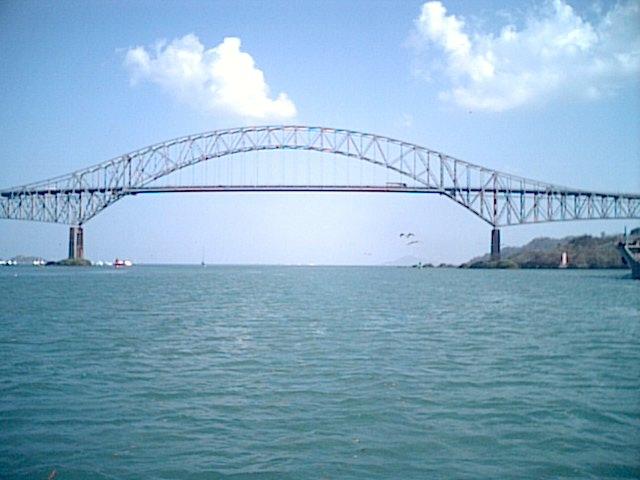The photo captures a massive, curved bridge arching gracefully over a strikingly blue, turquoise-hued body of water, which could be a lake, river, or ocean inlet. The bridge, featuring cross-hatched iron bars for stability, spans horizontally from left to right, connecting two pieces of land on either side. The right side hosts lush trees, and a boat appears to be approaching the bridge. In the distance, on the far left, more land is visible. The sky above is a brilliant blue, accented by two big, fluffy white clouds. Birds can be seen flying underneath the bridge, and faintly in the background, there is a hint of a mountain. Waves ripple across the water's surface, adding to the dynamic feel of the scene. Additionally, a vehicle is seen crossing the bridge, contributing to the sense of scale and activity in the image.